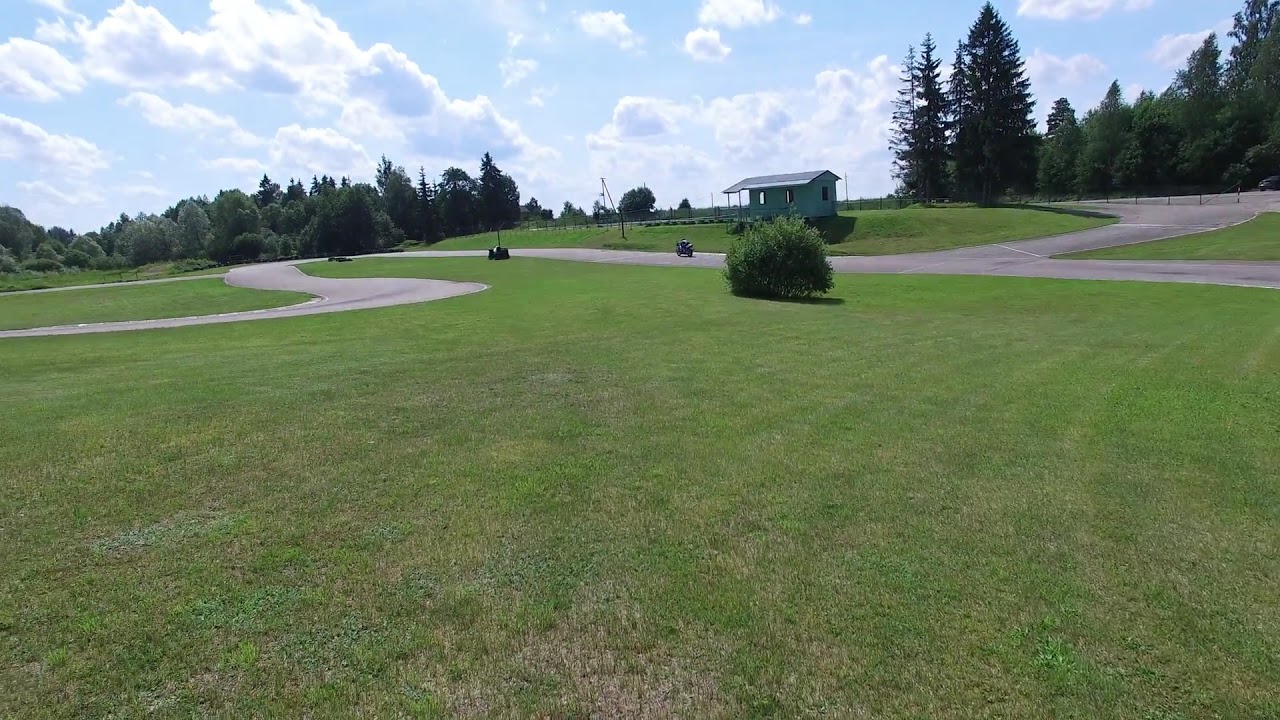This detailed digital photograph captures a sunny day with a bright blue sky adorned with high, puffy white clouds. The scene encompasses a picturesque setting that's likely a golf course or a park, featuring a winding blacktop path—colored blackish-gray—that traverses lush green fields and fairways. The pathway gracefully splits into three different directions and is surrounded by a variety of trees, including pines and other assorted species, creating a verdant canopy. There is a small greenhouse or building perched on a hill in the middle of the image, providing a charming focal point amidst the greenery. Along the main winding path, there appears to be a motorcycle or perhaps a golf cart heading west. The entire landscape is both serene and vibrant, with the sun casting a bright, inviting light across the scene, accentuating the abundant natural beauty of the setting. Additionally, a fence, bushes, and the intricate network of paths add depth and structure to the tranquil backdrop.